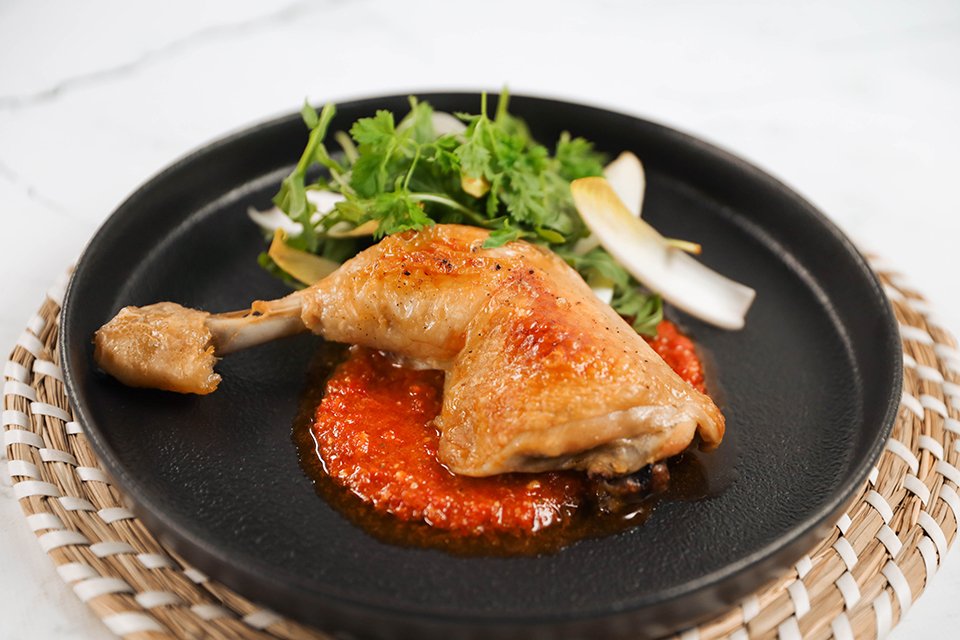This image, likely taken indoors for a restaurant promotion, features a meticulously arranged dish set against a minimalist backdrop. The photo displays a black plate, reminiscent of cast iron, resting on a beige straw mat with interwoven light white and tan fibers, placed on a sleek marble tabletop. The focal point of the dish is a succulent grilled chicken thigh and leg, presented atop a rich red chili paste. The chicken is artfully garnished with vibrant green cilantro and other greenery, including potential onions or leeks. Adjacent to the chicken, at the rear of the plate, lies a fresh spring salad, adding a burst of green contrast to the composition. The background remains unobtrusive, ensuring full attention is drawn to the elegantly plated food.